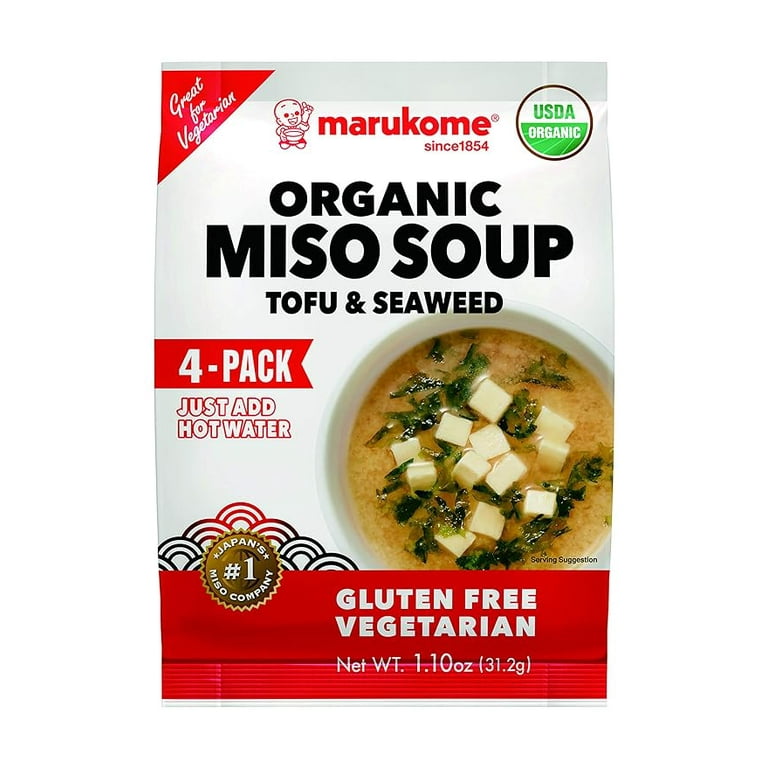This is the front of the Marukome organic miso soup package, prominently featuring its clear and minimalistic design. The package showcases a photograph of a white bowl filled with brown, cloudy miso soup, generously dotted with cubes of tofu and pieces of seaweed. A red triangular banner at the top left boasts "Great for Vegetarian" in white text. Adjacent to this, Marukome's logo—a cartoon baby holding up a finger, symbolizing "Japan's number one miso company"—is displayed proudly. The brand name "Marukome" along with the founding date "since 1854" is also featured near the top. On the top right corner, a black circle outline houses the USDA organic certification mark. Below, bold black text reads "organic miso soup tofu seaweed," emphasizing the key ingredients. The package includes a red banner at the bottom stating "gluten-free" and "vegetarian" in white text, and indicates the net weight of 1.10 ounces (31.2 grams). Additionally, the packaging highlights that this is a four-pack, with instructions to simply add hot water.